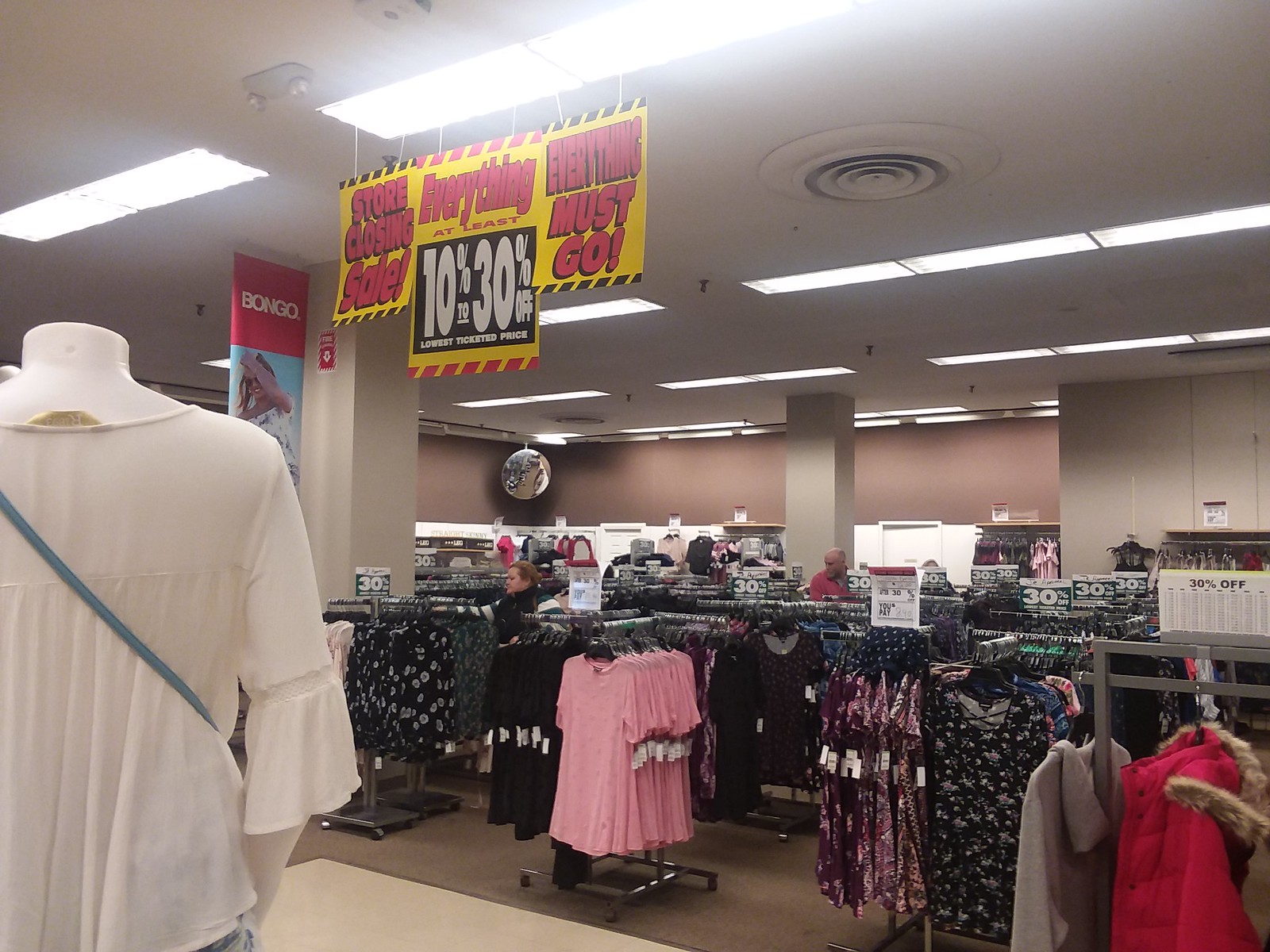This color photograph captures the women's section of a department store, which is currently having a store-closing sale. Multiple fluorescent light fixtures and fire sprinklers hang from the ceiling, along with a prominent sign that reads, “Store Closing Sale. Everything Must Go. 10-30% Off.” The sign has a yellow background with red writing, and the discount details are highlighted with a black background and white text. 

Below the sign, there are numerous racks filled with various clothing items, including pink, purple, and blue dresses, as well as shirts in solid colors and floral patterns. A few racks display banners offering 30% off, and tags indicating discounts can be seen above the clothing. The store features a brown carpet that transitions into a white tile floor, adding to the visual distinction between sections. To the left, a blue and red "Bongo" sign hangs from the ceiling, and a mannequin dressed in a white shirt with a blue purse is also visible. A brown wall provides a backdrop to the scene, and a few shoppers can be seen browsing through the sale items.